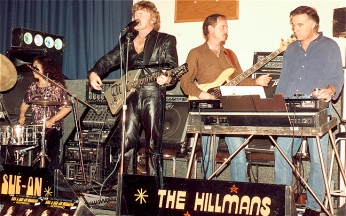This image captures a vintage scene of the band "The Hillmans" performing on a soundstage. The photograph, slightly out of focus and suggesting a mid-70s era, has a horizontal rectangular orientation. On the far left, a woman with short sleeves and a floral top paired with black pants is seated, playing drums. Just a few inches to her right, a man in a black leather outfit, consisting of both a jacket and pants, stands playing a greenish-colored guitar. He sports a mullet hairstyle with brown hair and sandals. Slightly behind him towards the center, another man in a long-sleeved brown shirt with blue jeans and a brown mustache is also playing a guitar. On the far right, a man with graying hair, wearing blue jeans and a blue button-down shirt, is playing an old keyboard.

The background features a combination of a dark blue curtain on the left side and a white wall toward the center and right. At the bottom of the stage, there are two signs, one prominently displaying the band’s name "The Hillmans" in yellow vintage print on a black background, and another partially visible sign that seems to spell "Sue Ann." The equipment and the musicians' attire, along with the overall ambiance, hint at a nostalgic, retro vibe, with the instruments and the sign contributing to the dated aesthetic.